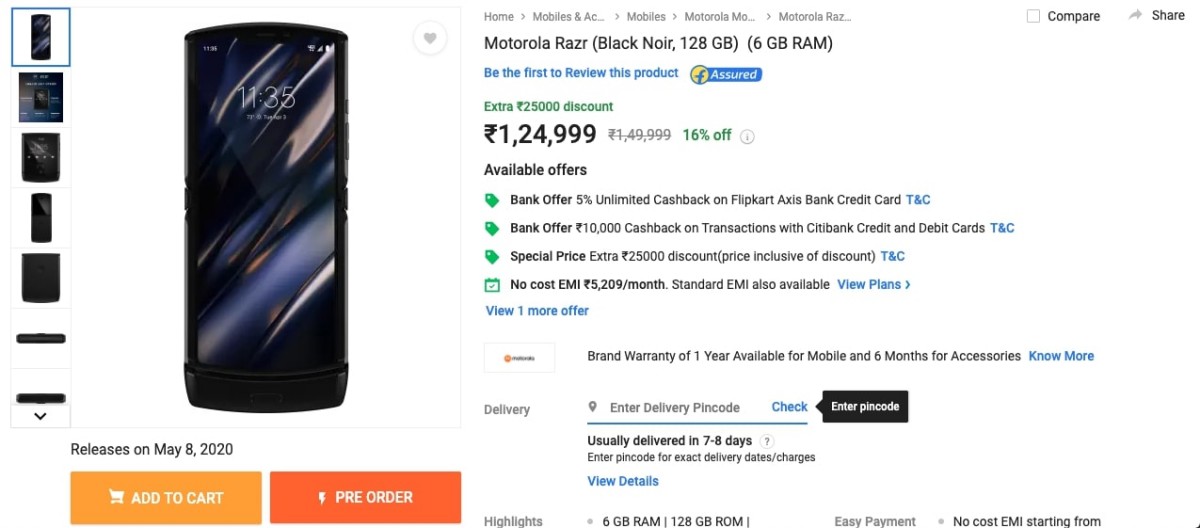This screenshot from a mobile phone website is a detailed display page for the Motorola Razr. On the left, there are eight vertically stacked images showcasing the smartphone from various angles, including close-ups from the side, back, right, and left. To the right of these images is a prominent full-screen shot of the cell phone's front, highlighting its black bezels and side buttons. The phone's screen displays the time in white text on a black and grayish background. Beneath the screen, a thin gray line features the release date: "Release on May 8, 2020."

Below this line, there are two buttons: a light orange button labeled "Add to Cart" and a dark orange button with a lightning bolt, labeled "Pre-order." Adjacent to these buttons, a dedicated text box provides more information about the phone. The top of the text box includes navigation headers reading "Home," "Mobiles," and "Motorola Razr." On the far right of these headers is a checkbox labeled "Compare," accompanied by an arrow labeled "Share."

Further down, the text box details the phone's specifications: "Motorola Razr (Black Noir, 128 GB, 6 GB RAM)." Additional information includes a prompt to "Be the first to review this product," followed by the price: "$1,124.99." The section also highlights available offers and special bank offers. Warranty information for the phone is also provided further below. This comprehensive layout affords potential buyers detailed insights and options straight from the mobile shopping interface.